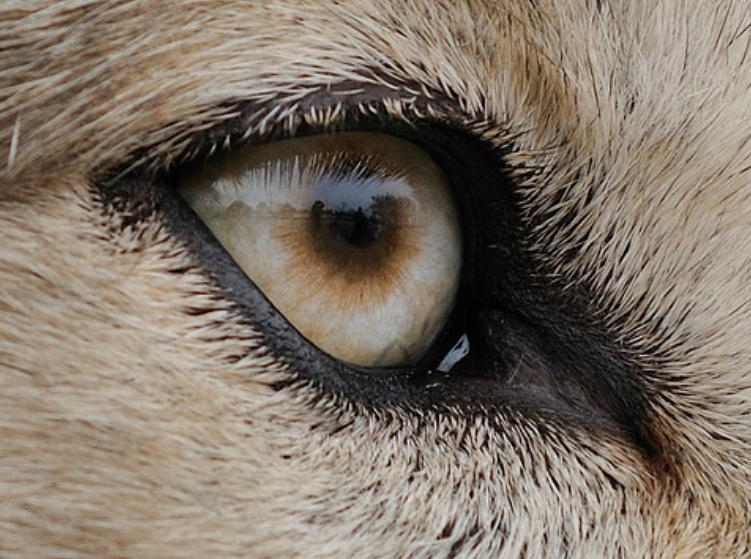This photograph is an extreme close-up of an animal's eye, likely a dog or possibly a wolf, with a stunning level of detail. The eye itself features a light greenish-brown iris with a brown circle around the black pupil, giving it an almost pearl-like or hazel appearance. Surrounding the eye, the skin is black, and the tear ducts are also black and appear wet. The fur around the eye is a sandy, beige-brown color, with short, individual strands clearly visible. Reflecting in the animal's calm eye, you can discern vague shapes of multiple people and trees, hinting at a possible outdoor environment. The intricate details, from the black eyelids to the mixed-colored fur, suggest a detailed portrait of a serene and possibly domesticated animal.